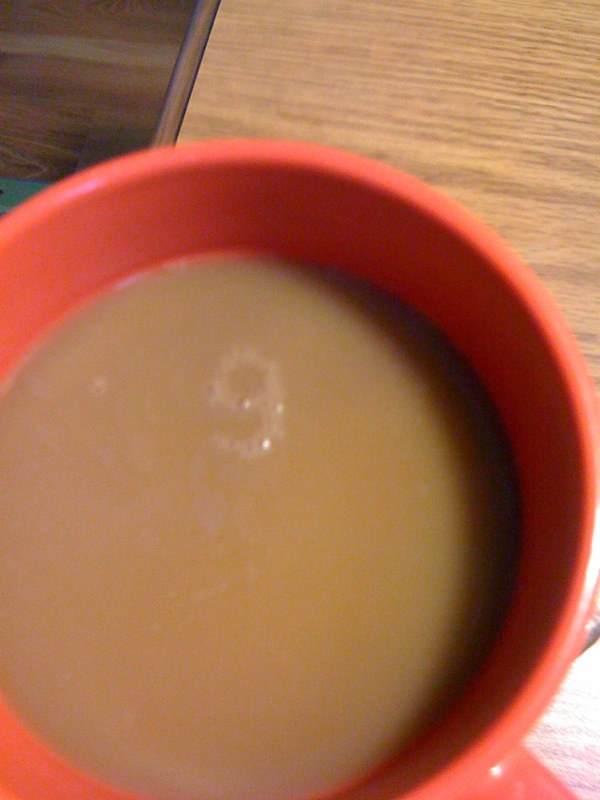This image is a color snapshot taken from above, looking directly down into a light red or red-orange coffee mug, which fills up four-fifths of the frame. The photograph is slightly out of focus, especially towards the lower part, likely due to a close-up attempt that didn't quite adjust properly. The surface on which the coffee mug rests resembles faux wood, possibly Formica styled to look like real wood, suggesting it could be a teacher's desk or similar. Inside the mug, there's a milky coffee or tea with bubbles clustering in an unintentional yet distinct shape of the number nine. In the background, part of the wooden desk and a section of a wooden floor with a small green patch peeping out are visible, though details about the green element remain unclear. The top half of the image is sharper, providing a clearer view of the formica desk and the mug's handle.